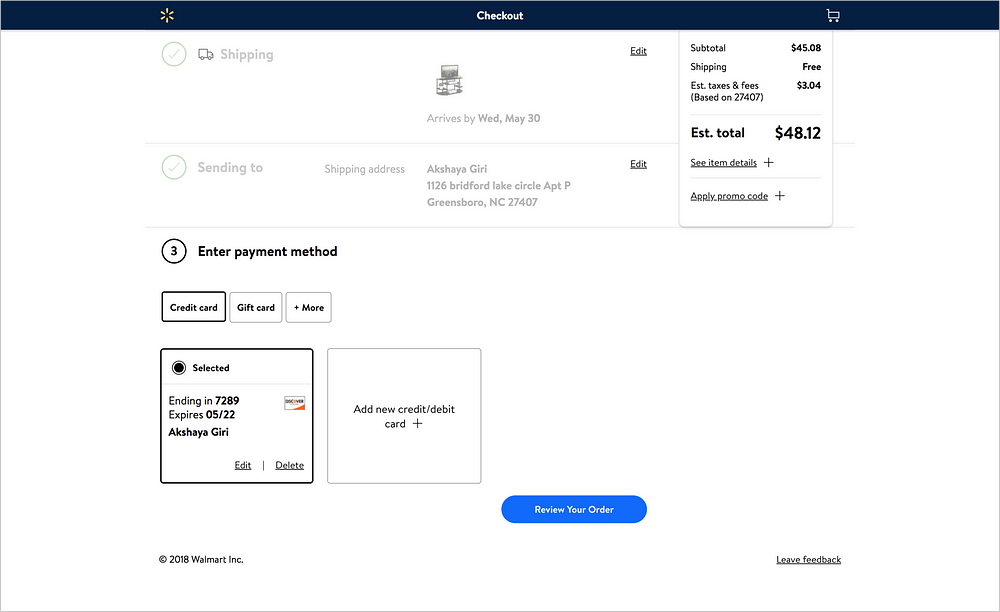The image depicts a Walmart checkout webpage. At the top of the page is a black bar stretching horizontally across the screen. In this bar, the Walmart logo is prominently displayed on the left, while the word "Checkout" is situated at the center in white text. On the far right of the bar, there is a shopping cart icon.

Below the black bar, the webpage is divided into several sections. The first section shows "Shipping and sending to" and "Enter payment." The "Enter payment" section is currently highlighted in black. On the right, a summary box displays the subtotal of $45.08, with free shipping, estimated taxes of $3.04, and an estimated total of $48.12.

In the payment section, users can choose their payment method. The image shows that the "Credit Card" option has been selected, indicated by a black-filled circle. The details of the selected credit card are visible: it ends in 7289, expires in May 2022, and is a Discover card belonging to Akisha Yairi. There are options to edit or delete the credit card information. Next to this, there is an unselected "Add New Credit/Debit Card" option with a plus sign, allowing users to add additional cards if needed.

At the bottom, there is a blue button with curved edges in the center that says "Review Your Order." To the right of this button, there is an option to leave feedback.